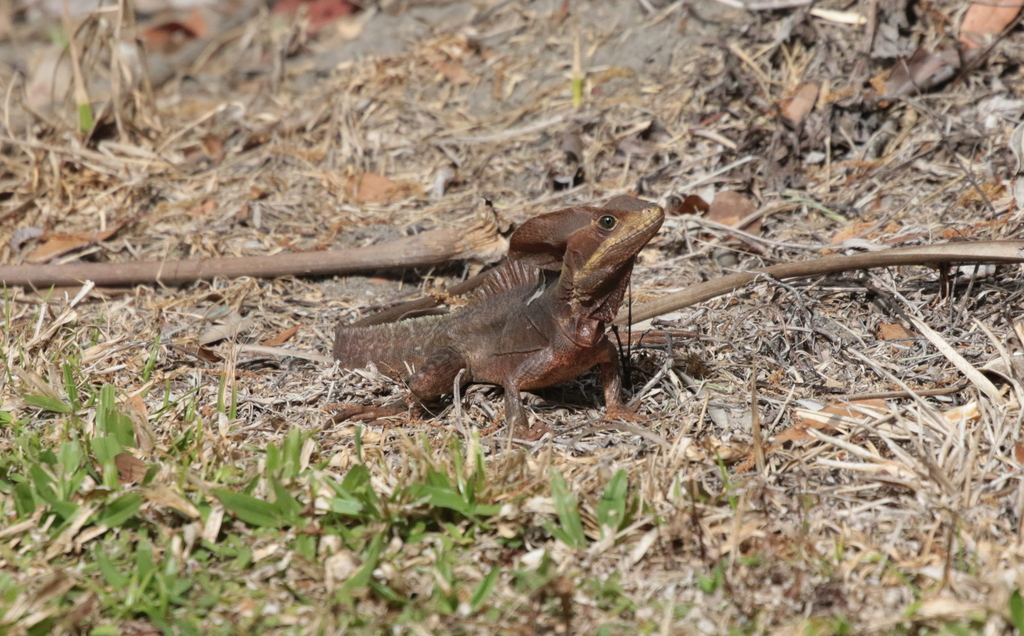The image captures a very small, dark brown lizard with a large crest on its head, giving it an almost dinosaur-like appearance. The lizard, which also exhibits a yellow mouth and black beady eyes, is looking up and appears to be soaking up the sun while standing atop a mix of debris that includes small sticks, dried leaves, and branches. The lizard's tail is curved, adding to its poised stance. Surrounding the lizard is a landscape dominated by dry, barren ground covered in dead, shrubby material and patches of dirt. In the foreground, a few blades of grass and some green leaves peek through the otherwise brown and desolate terrain. The top half of the image continues this theme of dryness, lacking any vibrant greenery, and suggesting an arid or sun-scorched environment.